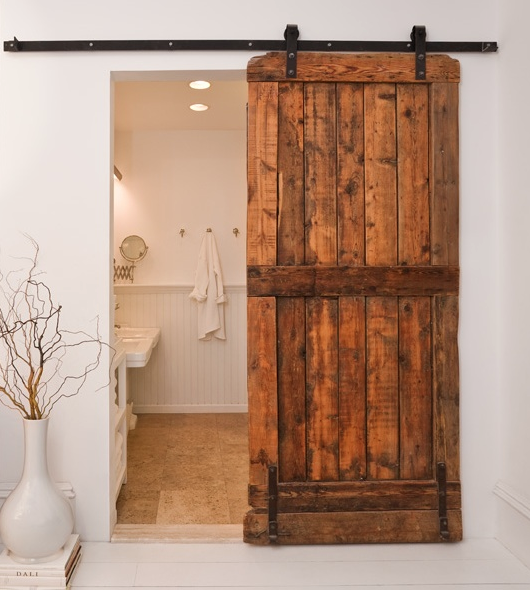This is a detailed color photograph of a bathroom, taken from an adjacent room. The prominent feature in the foreground is a weathered wooden sliding door that evokes a rustic, barn-like aesthetic. The door, constructed from horizontal and vertical wooden planks, is fastened with black brackets and hangs from a black metal bar that extends across the white wall above. The door is partially open, revealing the pristine, white-themed interior of the bathroom.

On the left side of the image stands a white vase containing brown branches, positioned on a cream-colored surface beside a stack of books, one of which features the letters "D-A-L-I." Inside the bathroom, directly visible, is a white wall adorned with three hooks, one holding a white towel. Beneath the hooks is white wainscoting, and the floor appears to be a brown tile.

The bathroom features two circular, recessed ceiling lights casting a white light. To the left, above one of the two white sinks, is a gold-colored circular mirror mounted on an extendable scissor arm. The overall ambiance of the scene blends rustic and modern elements, creating a clean and inviting space.